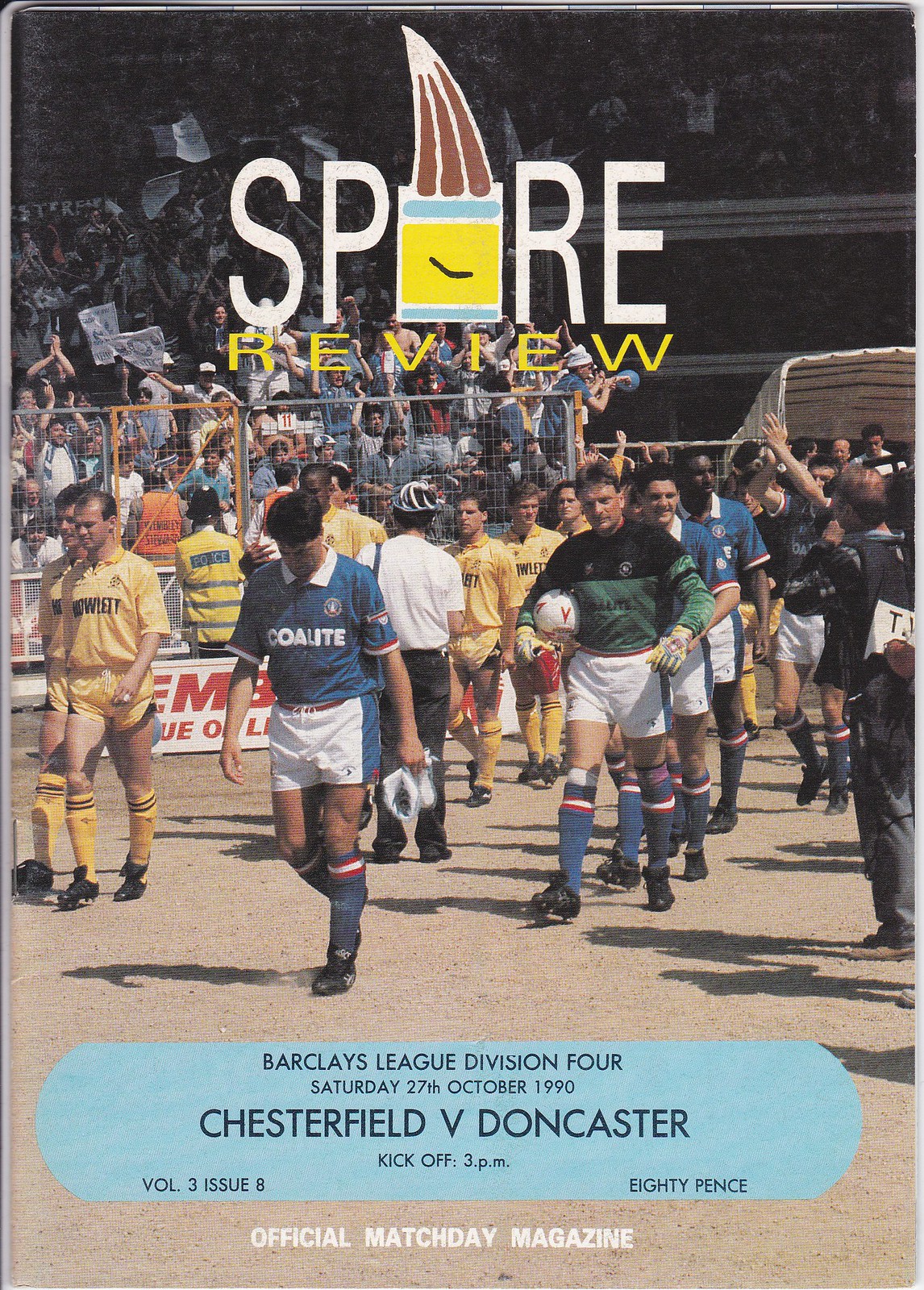The image is a rectangular program cover for a soccer match. At the top, it prominently displays the title "SPARRE REVIEW," with a logo that features a square clock with horns. Beneath this title is a detailed description of the football match information: "Barclays League Division 4, Saturday 27th October 1990, Chesterfield versus Doncaster, kickoff at 3 p.m." Additionally, it mentions "Volume 3, Issue 8, 80 pence" and "Official Match Day Magazine" printed at the bottom in white text on a blue band.

The photograph within the program shows several soccer players from two different teams preparing to start the game. One team wears blue and white kits, while the other team is dressed in gold uniforms. The goalkeeper is distinguishable in a green and black kit. Behind the players, the stands are filled with enthusiastic fans waving signs and cheering, all situated behind a barrier. The colorful crowd adds vibrancy to the image, encapsulating the anticipation and excitement just before the match begins.